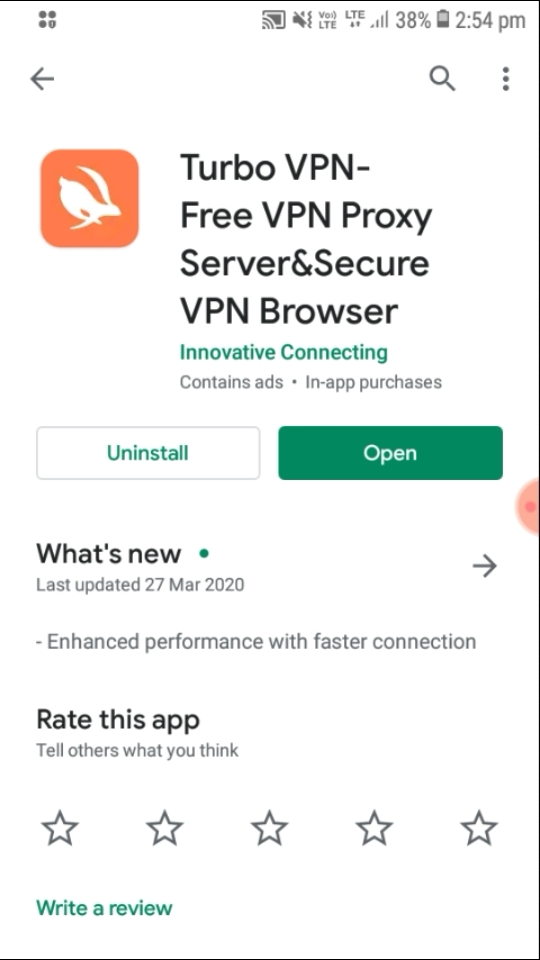Screenshot of an app store interface showing the TurboVPN app. At the top right, the status bar displays various icons including a cast TV icon, a ringer icon, two data icons, and a battery icon showing 38% charge. The time is 2:54 PM. Below the status bar, the interface features a left-pointing arrow on the left side, and a search icon followed by three vertical dots on the right side. The app section centers on TurboVPN, described as "Free VPN Proxy Server & Secure VPN Browser, Innovative Connecting" and notes it contains ads and offers in-app purchases. On the right, a green button says "Open," and a white button on the left says "Uninstall."